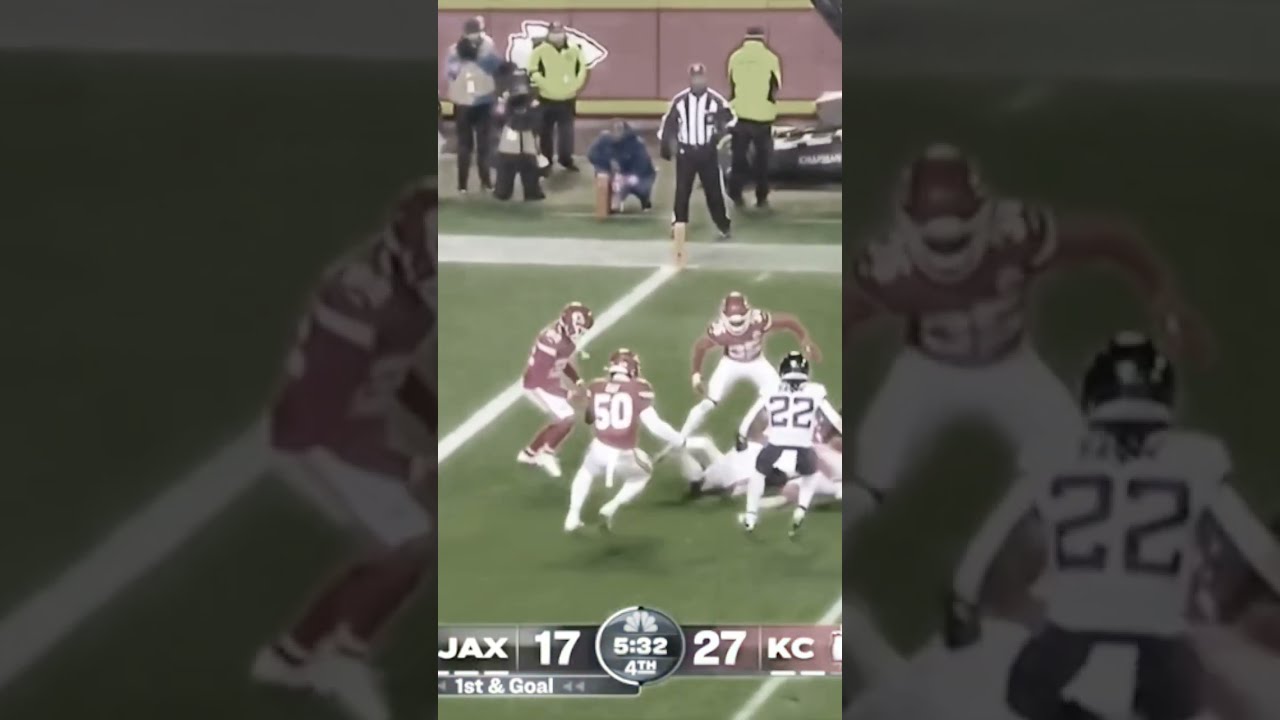The image is a detailed, horizontally rectangular composition divided into three panels. The left and right panels are darker and less detailed, displaying closer views of the central image. The central, lighter panel is superimposed over the darker panels, creating a clearer, more detailed depiction of an NFL football game between the Jacksonville Jaguars and the Kansas City Chiefs. 

In the left panel, you see a partially cut-off profile of a football player in red, facing right, with the goal line and end zone behind him. The central panel, brighter and more vivid, features an action shot showing three Kansas City players in red, numbers visible, converging on a play. The Jacksonville player in white, number 22, is visible to the right side, with another player being tackled in the middle. The background includes a referee standing on the goal line and several spectators, some more lifelike and others appearing drawn-in. 

A black band at the bottom of the image displays game information: Jacksonville leads with 17 points, Kansas City with 27, with 5 minutes and 32 seconds remaining in the fourth quarter, and it's first and goal.

The right panel shows a close-up of a Kansas City player in red, facing forward and ready to tackle, with the number 22 Jacksonville player positioned at the bottom right, his back to the viewer. Overall, the composite image effectively captures a dynamic and detailed moment from the football game.